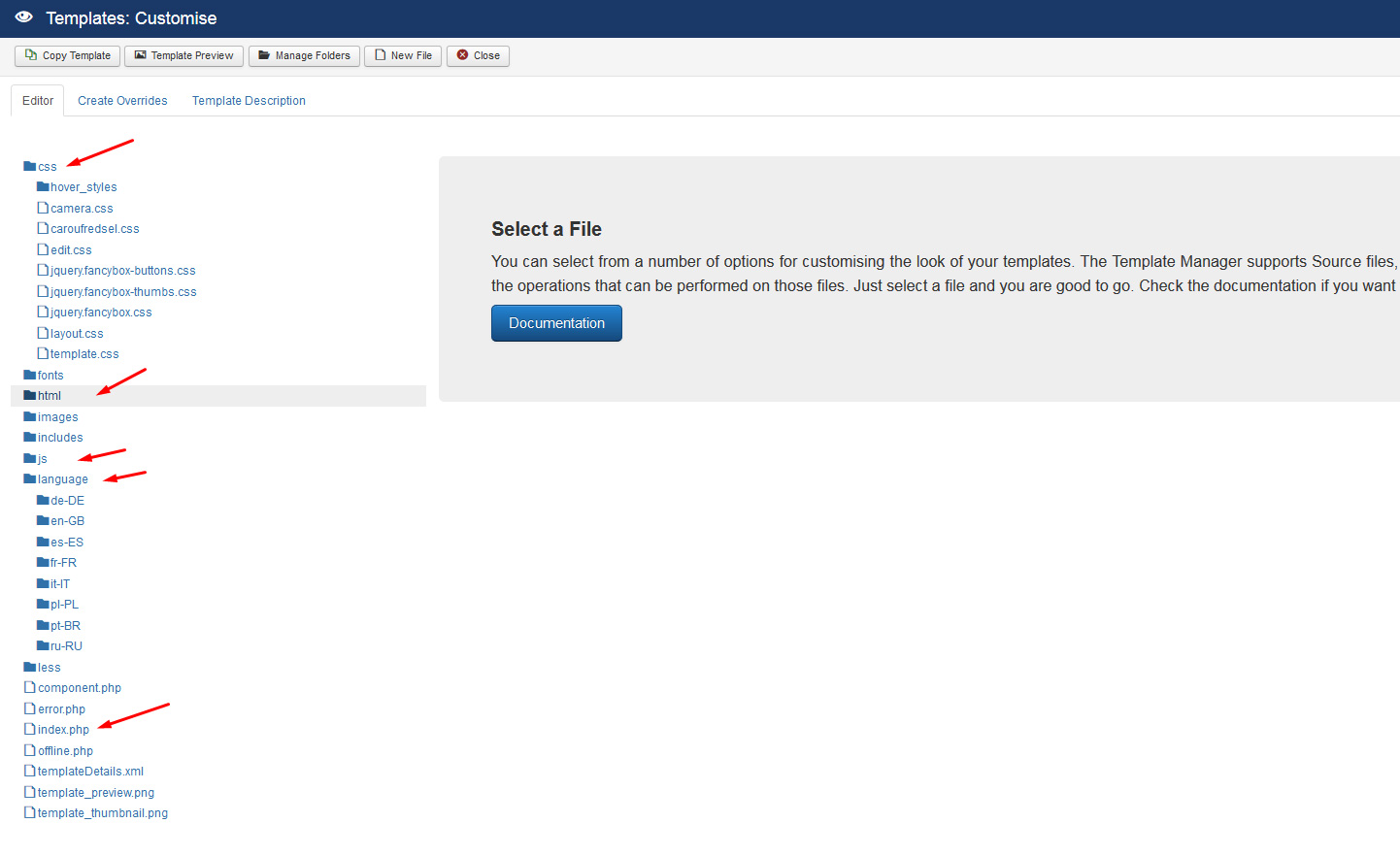In this detailed image, we see a user interface with various elements related to template customization and file management. At the top, a long blue rectangle with the label "Templates" is visible, accompanied by a small "i" icon on the right-hand side. Below that, there are several functional options listed: "Customize," "Copy Template," "Template Preview," "Manage Folders," "New File," and "Encodes."

Further down, the interface displays an "Editor" section with options such as "Create Overrides" and "Template Design." A red arrow is pointing towards an area labeled "CSS," next to which there are several blue folders and other file icons. The first blue folder is labeled "Hover Styles," and beneath it is a white document icon labeled "Camera.CSS."

Continuing the list, we see:
- "CAROUFREDS.EL.CSS"
- "Edit CSS"
- "JQuery Fancy Box Button CSS"
- "JQuery Fancy Box Thumbs.CSS"
- "JQuery Fancy Box.CSS"
- "Layout CSS"
- "Template CSS"

Next is a series of blue folders categorized by typography and content types:
- "Fonts" (blue folder)
- "HTML" (blue folder with a darkened appearance and a red triangle pointing to it)
- "Images" (blue folder)
- "JS" (blue folder with a red triangle pointing to it)
- "Language" (blue folder with a red triangle pointing to it)

Following this, we see language-specific folders:
- "DE" (German)
- "EN" (English)
- "ES" (Spanish)
- "FR" (French)
- "IT" (Italian)
- "PL" (Polish)
- "PT-BR" (Brazilian Portuguese)
- "RU" (Russian)
 
Underneath these language folders, we find several file icons:
- "component.php"
- "era.php"
- "index.php" (highlighted with a red arrow)
- "offline.php"
- "template_details.xml"
- "template_preview.png"
- "template_thumbnail.png"

At the bottom, a gray rectangle labeled "Select a file" provides instructions on customizing template appearances through the Template Manager, which supports operations on source files. It encourages the user to select a file and offers a blue button linking to "Documentation" for further assistance.